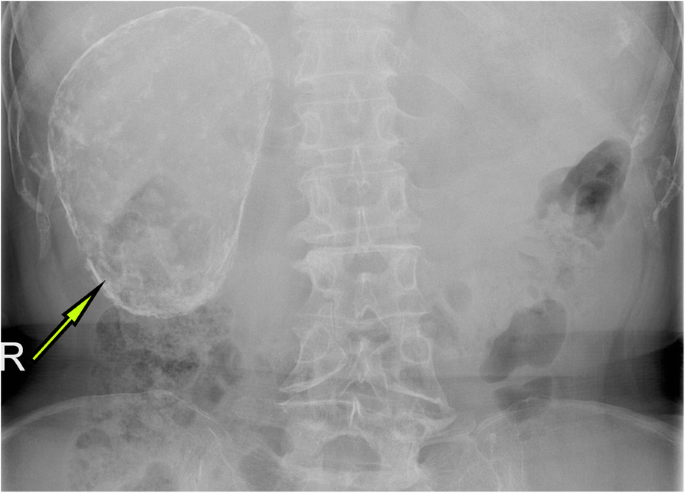This monochrome x-ray image of a human body prominently displays the spine, extending from the cervical to the lumbar vertebrae, though not quite reaching the neck. The ribs are faintly visible, appearing as protruding, cloudy shapes. The image also captures a section of the lower abdomen, including the kidney. Notably, a yellow arrow is superimposed on the x-ray, pointing towards an irregularly shaped mass on the left side of the image, which could be the right side of the body, depending on orientation. Adjacent to this arrow is a white letter "R," likely indicating the anatomical side being examined. The x-ray's ghostly, transparent quality allows for a detailed view of various structures, albeit some areas remain indistinct.